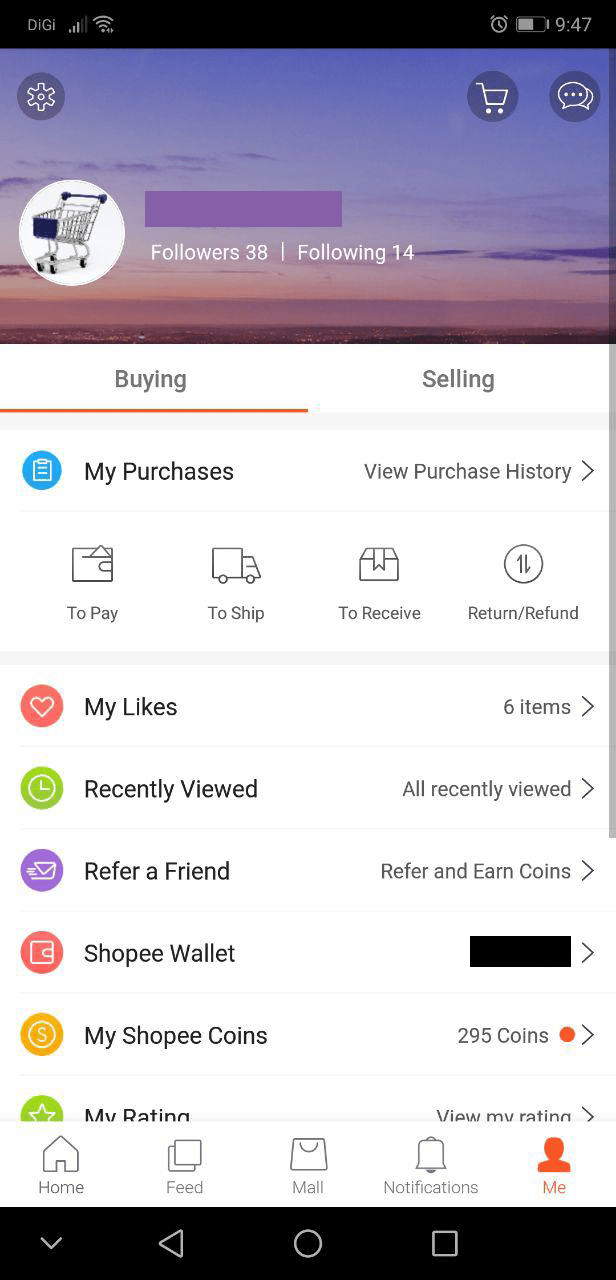A detailed image caption:

This image is a screenshot taken on a mobile phone, as indicated by the clock at the top right corner displaying the time as 9:47. Positioned to the left of the clock is a battery icon showing approximately 60% charge, and an alarm clock symbol is also visible. On the top left, the status bar shows the carrier name 'Digi' followed by signal strength with 3 out of 5 bars and a fully filled Wi-Fi icon.

The main background of the screenshot features a sky with a distinct purplish hue, creating a serene yet vibrant tone. Adjacent to this, there is a circular icon with a white background, showcasing a blue-colored shopping cart with both the front and the grip highlighted in blue.

To the right of this icon, the word "FOLLOWERS" is displayed, accompanied by the number 38, indicating the follower count. Similarly, the word "FOLLOWING" is shown with the number 14, signifying the count of profiles being followed.

Beneath these details are the words "BUYING" and "SELLING," with an orange line underscoring "BUYING" to possibly indicate it is currently selected. Below this, "MY PURCHASES" is listed to the left, with "VIEW PURCHASE HISTORY" to the right.

At the bottom of the image, there are four distinct icons each accompanied by descriptive text: "To Pay" (represented by an envelope icon), "To Ship" (a car icon), "To Receive" (a box icon), and "Return/Refund" (a coin icon). Each icon succinctly represents a different aspect of the user's transaction statuses.